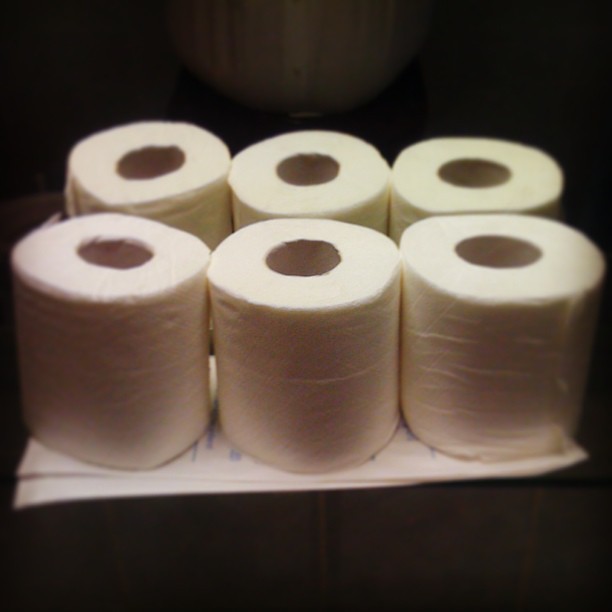This nearly square photograph features six untouched rolls of toilet paper, arranged in two tight rows of three across the middle of the image. Each roll is upturned, with the flat sides facing up and down, ensuring the central holes are visible. The rolls are densely packed together, touching one another as if they were arranged to fit snugly in a box. They sit on an unclear type of white paper that has some blue writing on it, resting on what appears to be a dark, partially visible surface, possibly a wooden table. The background is predominantly black, with a faint semi-circle of light above the central two rolls, casting the only hint of brightness in the otherwise dark scene. This light source transitions into a darker brown area, providing a subtle contrast against the black backdrop.